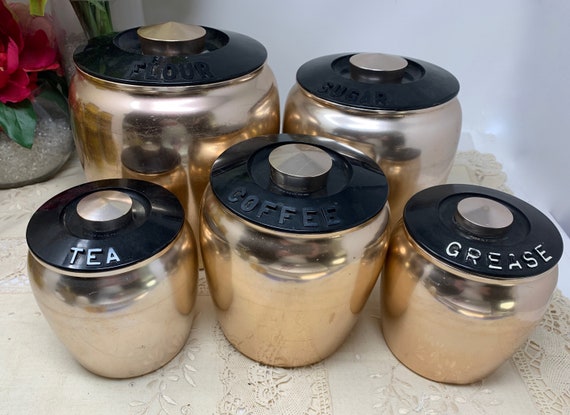The indoor photograph showcases a set of five metallic containers arranged on a light brown, intricately patterned tablecloth. These containers have a gold-bronze finish that reflects light, emphasizing their polished surfaces. Each container is topped with a matte black lid featuring a silver handle, and they vary in size, with two larger ones at the back and three smaller ones at the front. The labels on the lids identify their intended contents: the larger containers are marked "flour" and "sugar," while the smaller ones are labeled "tea," "coffee," and "grease." To the left of the containers, a glass vase with sand holds a vivid red flower and green leaves, adding a touch of natural color to the composition. The background is composed of a white wall, enhancing the contrasting colors of the containers and the table setting.